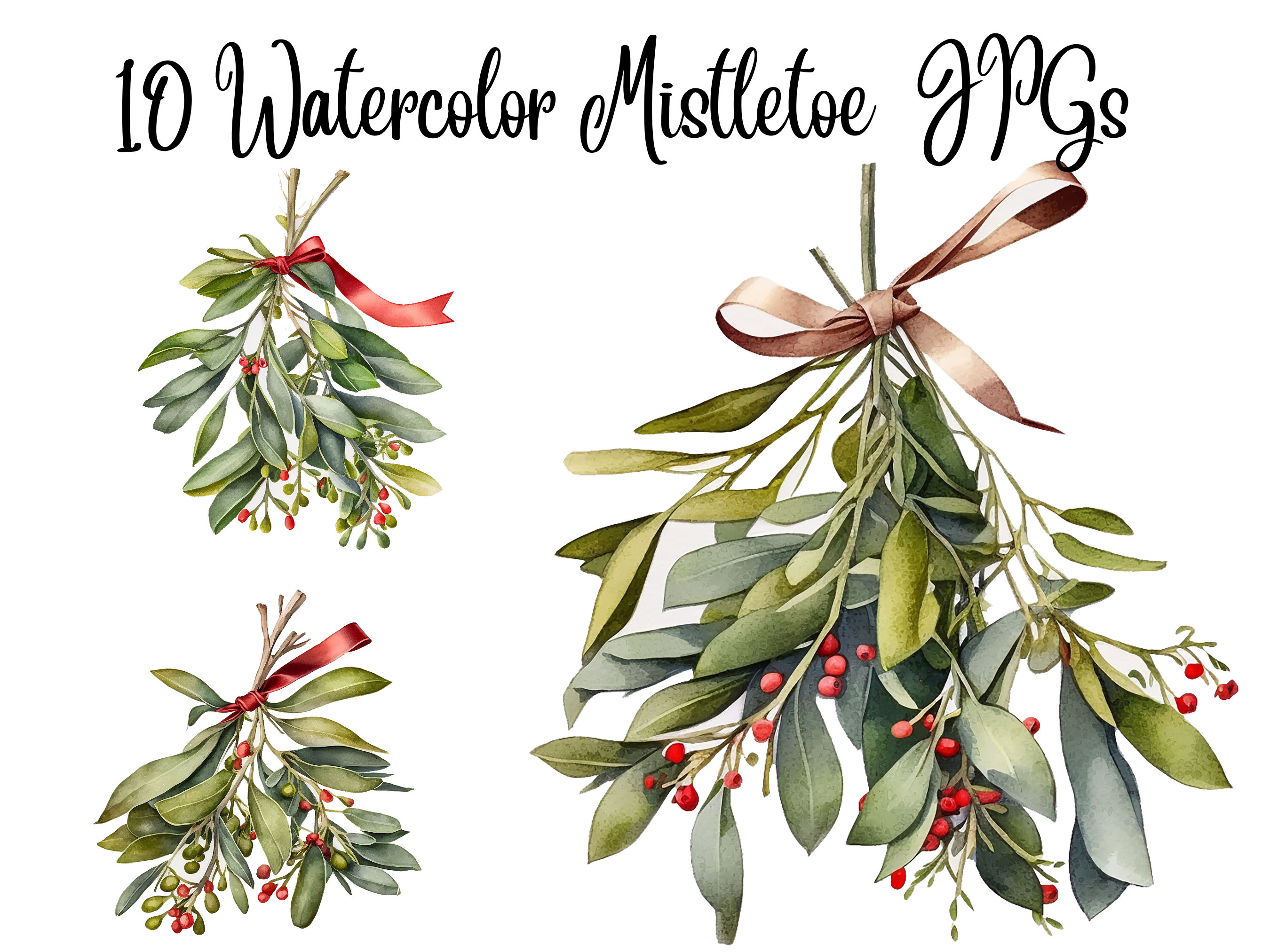The image features three digitally illustrated watercolor mistletoe bundles, each showcasing a distinct combination of light and dark green leaves with small, round red berries. The title "10 Watercolor Mistletoe JPEGs" is elegantly written in black cursive at the top. On the left, two smaller bundles are arranged vertically, with the top one tied with a vibrant red ribbon and the lower one appearing to lie more horizontally with varying shades of green. On the right, a much larger bundle presents a more natural and realistic appearance, with leaves that curl authentically and berries that stand out. This bundle is tied with a brown ribbon, adding a subtle contrast. The illustration captures the traditional holiday charm of mistletoe, complete with the festive allure of being kissed beneath it.